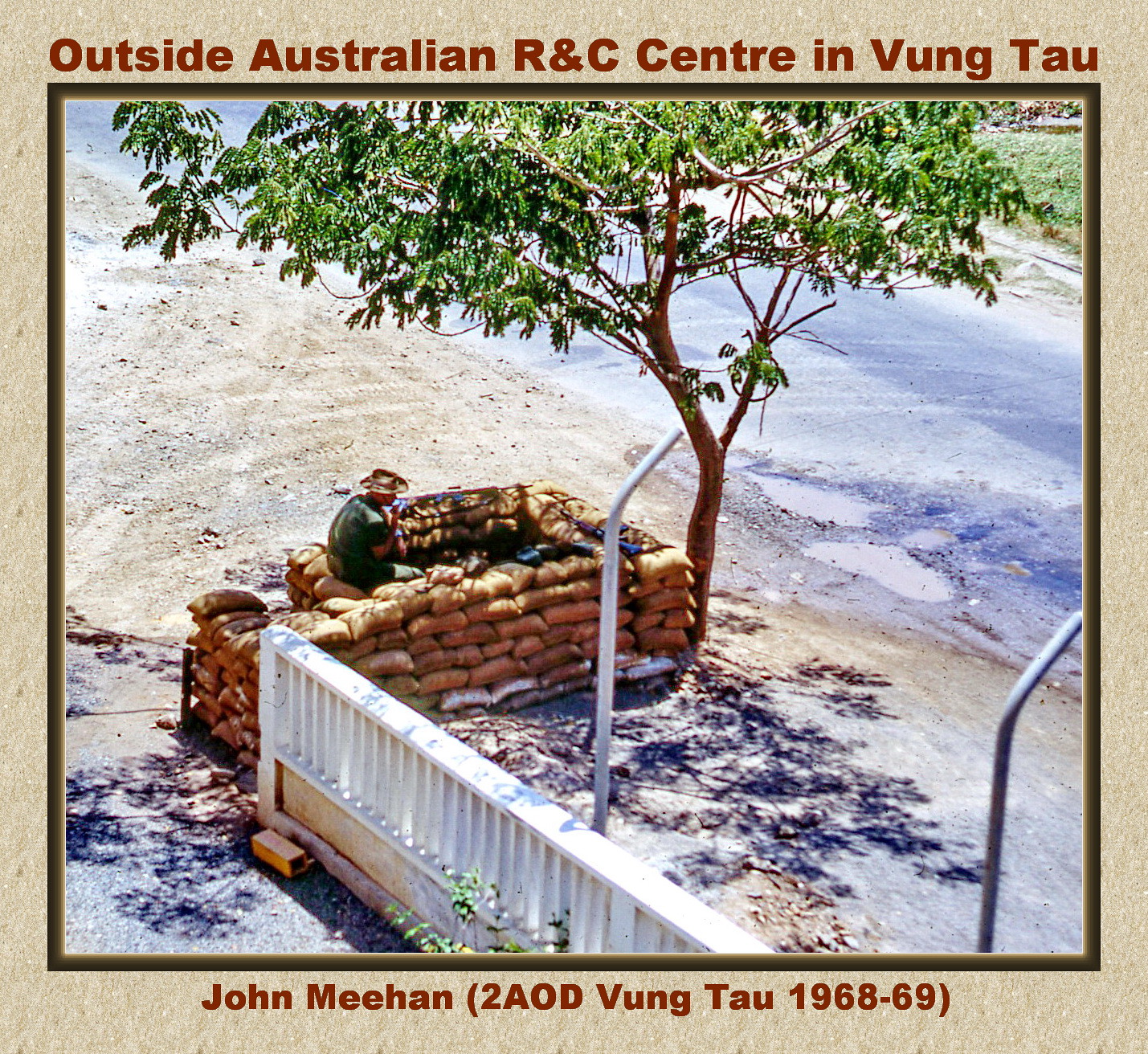The image depicts a color photograph taken outdoors during the daytime, featuring a man named John Meehan seated in a sandy area with a makeshift sandbag bunker surrounding him. This scene, set against a backdrop that includes a white fence on his right and a road on his left, is located outside the Australian R&C Center in Vung Tau. In front of the sandbag wall stands a tree, adding a touch of natural scenery to the image. The man, dressed in a brown safari hat and a green shirt, appears to be looking away from the camera. Text on the image indicates the location and time period: "Outside Australian R&C Center in Vung Tau" at the top and "John Meehan, 2AOD Vung Tau, 1968-69" at the bottom. The photograph has a border that frames the scene.